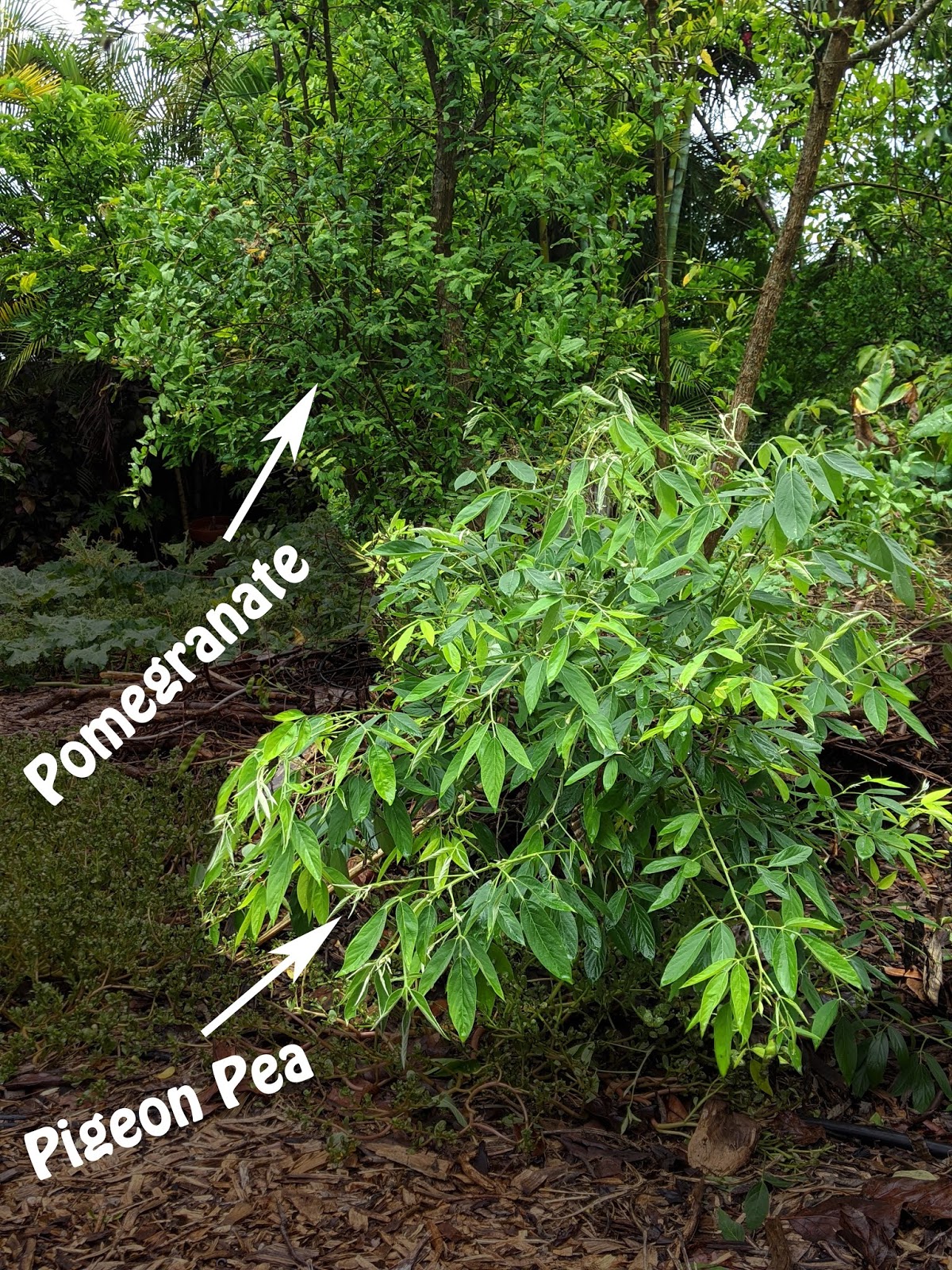The image showcases an outdoor scene with two distinct plant bushes, each labeled with a white arrow and text. In the foreground, a pigeon pea bush is highlighted with the label "Pigeon Pea" in white. Behind it, a pomegranate tree is similarly marked with the label "Pomegranate" in white. The pomegranate tree has multiple branches adorned with lime green leaves, and there is some sky visible with a few clouds in the upper right area. The ground is covered with brown mulch, comprising dried bark and twigs, and there's an absence of grass. The scene is well-lit, indicating that the photo was taken during daytime. In the backdrop, additional trees contribute to a lush, treed environment. No fruits are apparent on either the pigeon pea or pomegranate bushes, likely suggesting young plants that have yet to bear fruit.